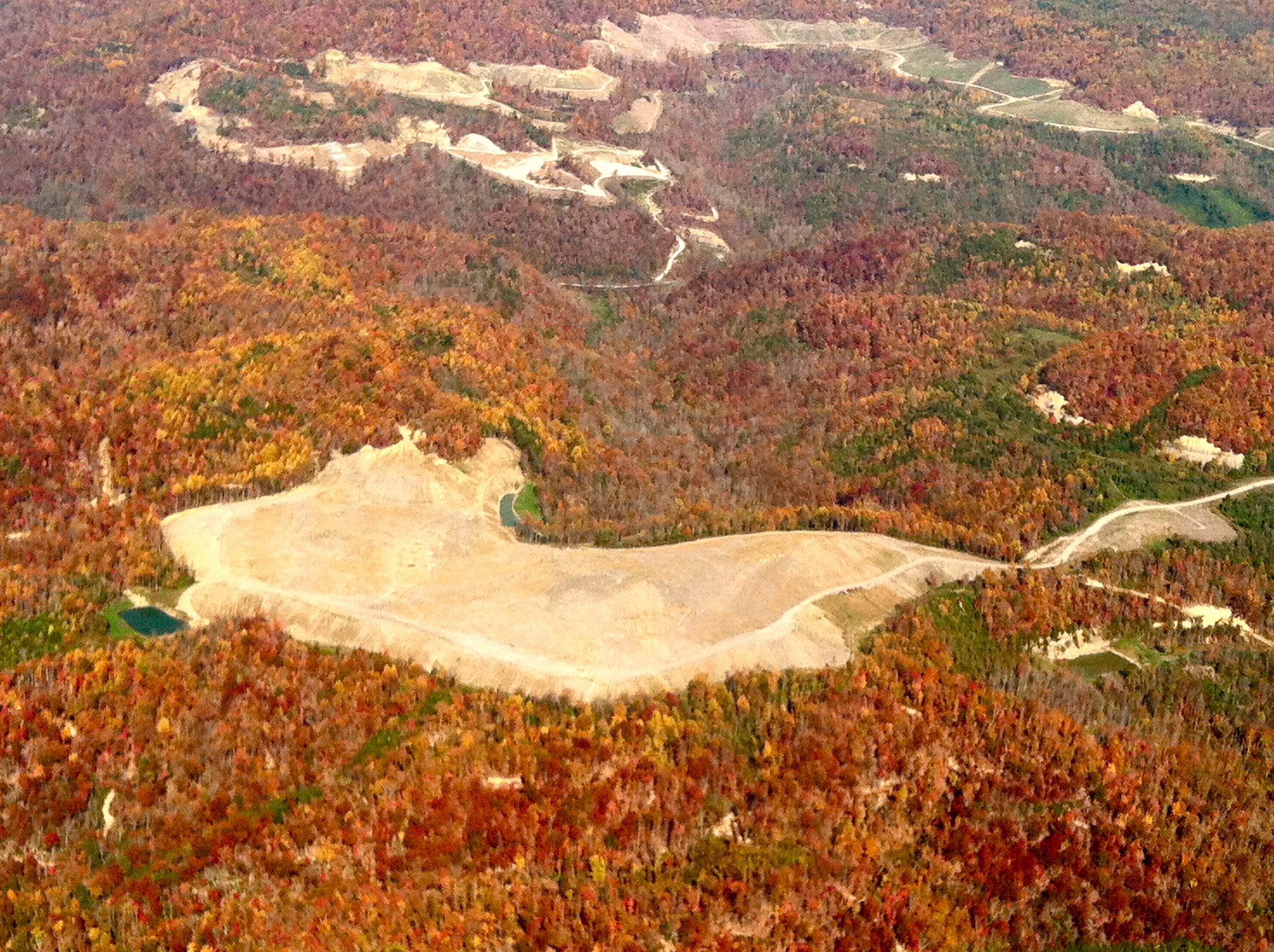This daytime aerial photograph captures an expansive, undulating landscape characterized by rolling hills and a diverse forest of vibrant fall foliage. Predominantly, the trees display rich hues of red, yellow, and orange, interspersed with patches of lingering summer green. The image reveals a large tract of land, possibly spanning hundreds or even thousands of acres. 

Amidst the forested areas are noticeable sections of bare land, distinguishable by their light brown, sandy appearance. These open spaces are crisscrossed by serpentine white roads, creating pathways through the colorful flora. In the far distance, additional bare land parcels are visible, suggesting the presence of residences, perhaps even mansions, evidenced by the faint outline of buildings. 

Despite the photograph's altitude, certain details like small bodies of water and the intricate winding of roads are discernible, contributing to the complexity and beauty of this autumnal terrain.